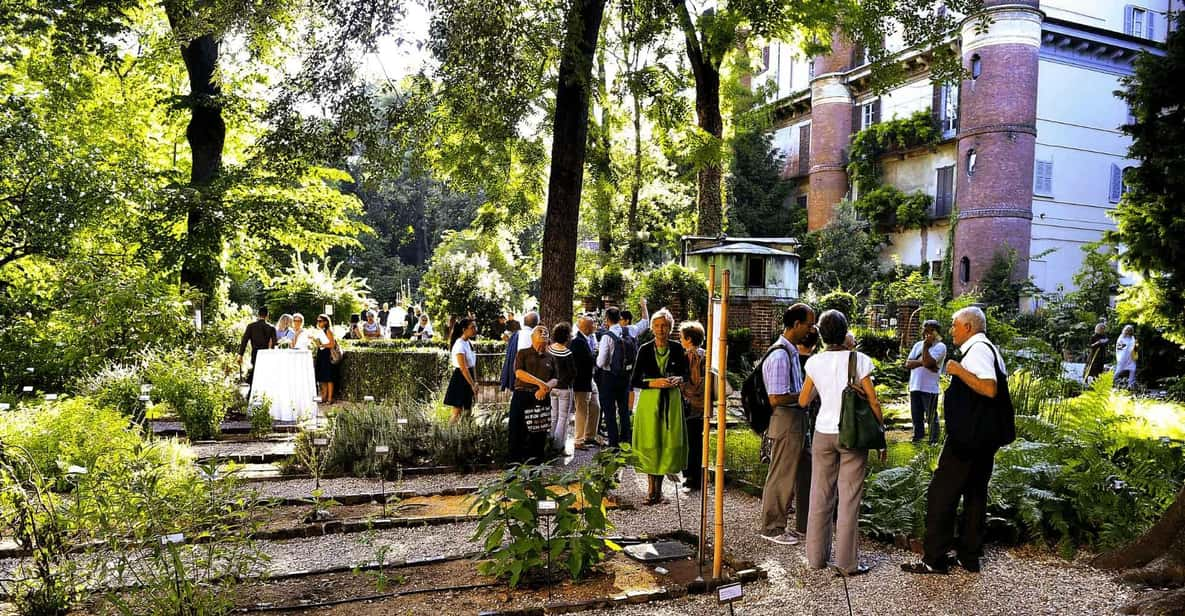This photograph captures an outdoor scene set in what appears to be a botanical garden or nursery. In the foreground, orderly rows of walkways made of gravel weave through various plots filled with plants, shrubs, and small trees, each accompanied by tiny signs with white cards describing them. Scattered throughout the garden are people standing either singly or in small groups, engaging in conversation. Many of them are dressed in business casual attire and carry backpacks or shoulder bags. The background reveals more people gathered around high-top tables draped in white tablecloths, participating in what appears to be a social or business event. Beyond the garden area, a large structure composed of white stone and red brick stands prominently, adorned with vines on its side, while an array of trees provides a lush backdrop.